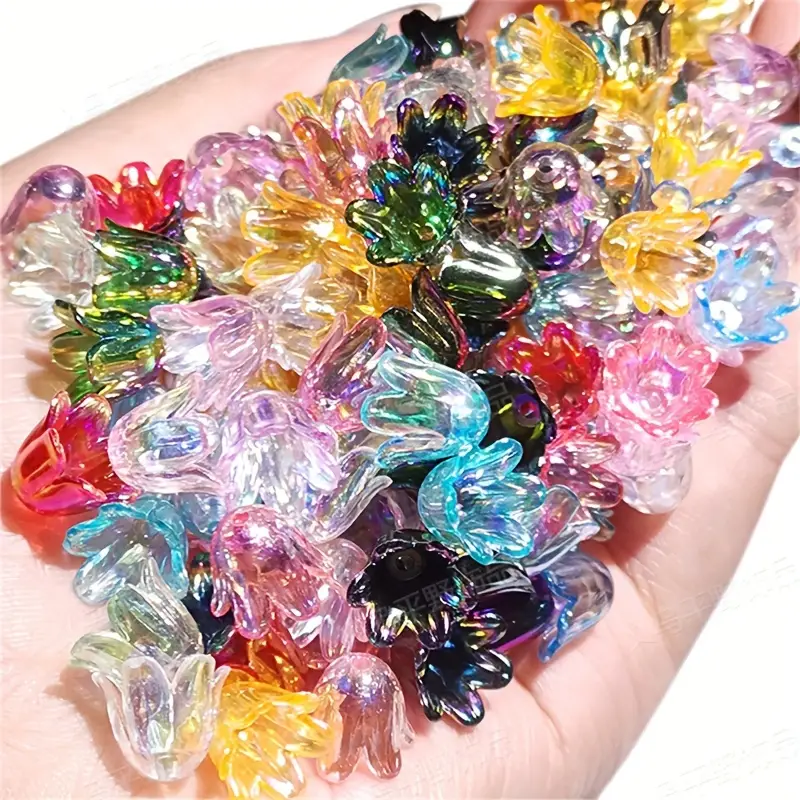In the image, a left hand is shown, its palm open and holding an assortment of small, glass-like or plastic floral items. These items resemble tulip-shaped flowers, with a translucent and colorful appearance, including shades of yellow, blue, pink, red, green, black, and a hint of silver. The items are intricately detailed, see-through with a tint of color, and are jumbled together, pointing in various directions. This gives the impression that the hand is grasping as many as it can fit, and the detailed lines and nails of the hand are clearly visible. The myriad of flowers, around 30 in number, create a vibrant and chaotic bouquet-like display within the hand.